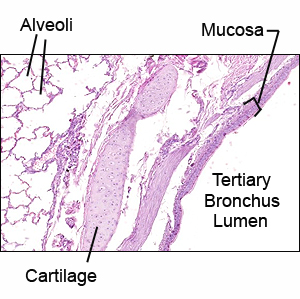The image is a detailed artistic rendering set within a black-outlined white rectangle, featuring abstract splotches and veins in shades of purple against a white background. The diagram, which appears to mimic a medical illustration rather than an actual slide, labels four specific anatomical features: alveoli, cartilage, mucosa, and tertiary bronchus lumen. These labels are marked in black, providing clear identification amidst the otherwise uniformly purple artwork. The illustration, devoid of any other colors or text, seems to be a simplified yet informative representation, potentially for educational use in a medical or science context. The overall impression is one of an abstract, yet structured depiction of respiratory system components.